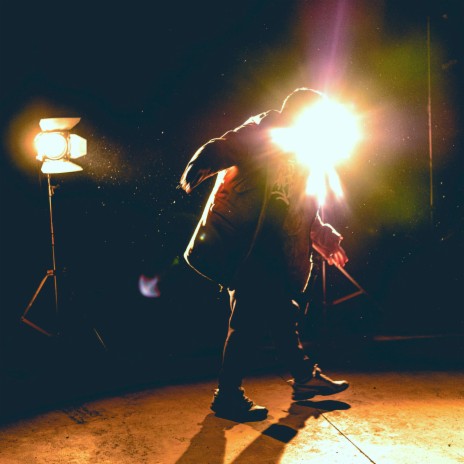The image features a man standing on a stage, illuminated by two powerful stage lights—one on his left and one on his right, with his head positioned right next to the right-side light, creating an almost silhouetted effect that obscures his face. The stage lights cast an orangish-brown hue over the scene, making the background difficult to discern except for a small, bluish-whitish stream of light with three distinct points visible to the left of the man. He is dressed warmly in a long winter jacket, jeans, and sneakers, and appears to be wearing a black shirt with white writing, though the text is not clearly visible. The man stands with his hands at his sides, focused downward, suggesting he is engaged with something on the ground. The overall color palette of the image includes shades of white, black, blue, and purple, with a predominately black background indicating the back of the stage.